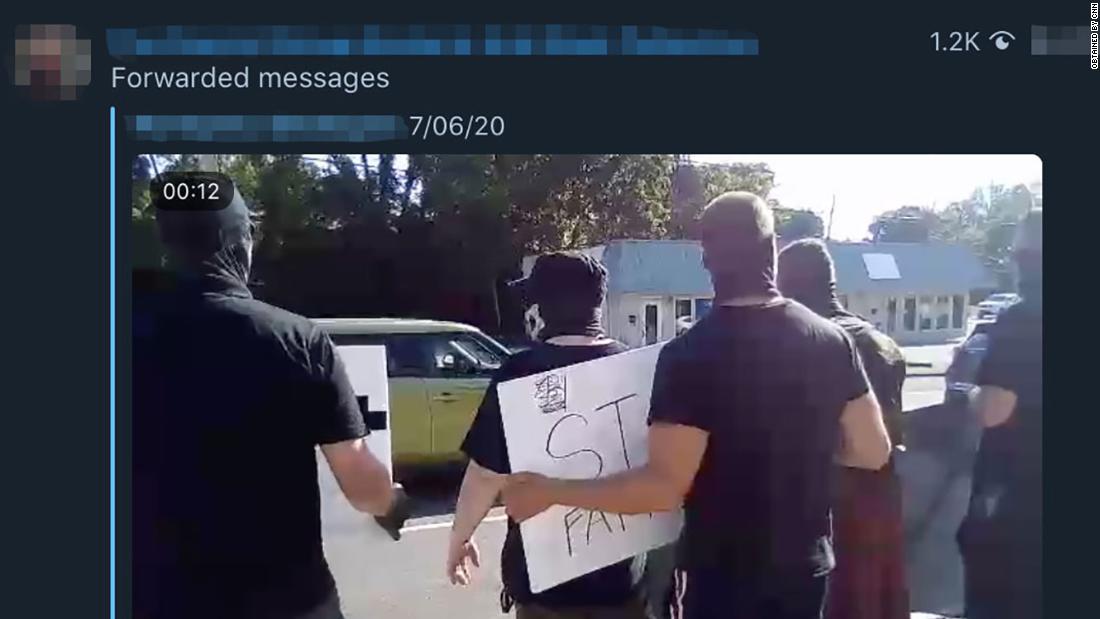A screenshot of an unidentified social media page features a centrally-placed video within a black background. The video, with a length of 12 seconds, is labeled at the top with the date "07/06/20," indicating it was posted on July 6, 2020. Above the date, the phrase "forwarded messages" is prominently displayed in white letters, suggesting the video has been shared from another source. In the top right corner, the video has accrued 1.2K views, marked by an eyeball icon.

The video itself shows the backs of five men, presumed to be white based on their visible arms, all donning black t-shirts, black masks, and facing away from the viewer towards a street. Some of the men are holding signs, the messages on which are obscured due to their positions. The men appear to be part of a group, possibly trying to conceal their identities. In the background across the street, there is a white building with a blue awning and some visible trees.